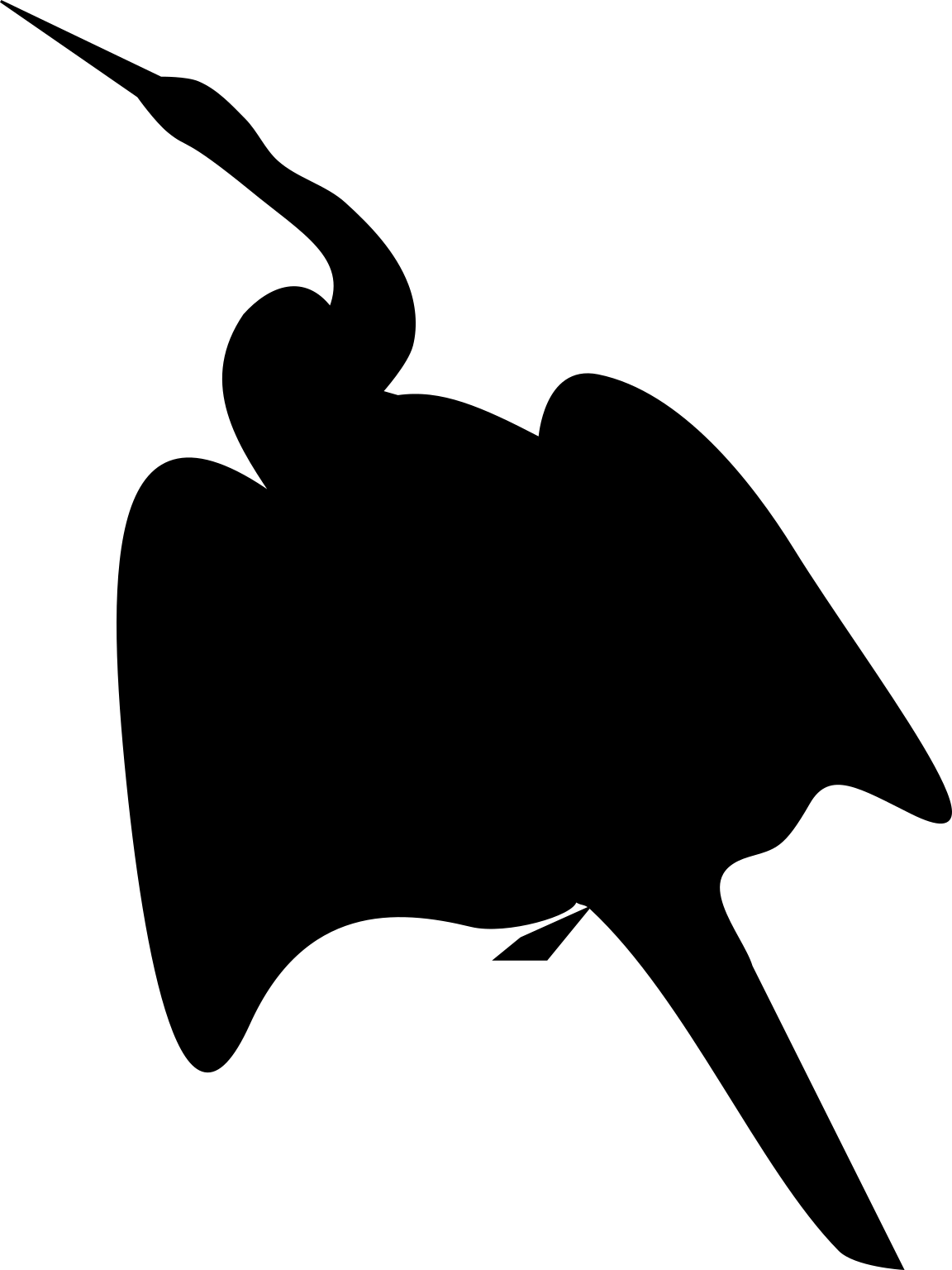This illustration features a simplified black silhouette of a bird, likely a stork or similar species with a long, sharp beak and an elongated neck. The bird is positioned on a pure white background, making the contrast striking. Its neck curves intriguingly, attaching to an oval body from which two wings extend. The head, located at the upper left corner, suggests an upward flight direction. Additional details include a stylized foot, a small pointed tail, and a narrow head with a pointed beak. The minimalistic, inkblot-style drawing contains no shadows or text, evoking the kind of imagery that might be used in psychological evaluations.